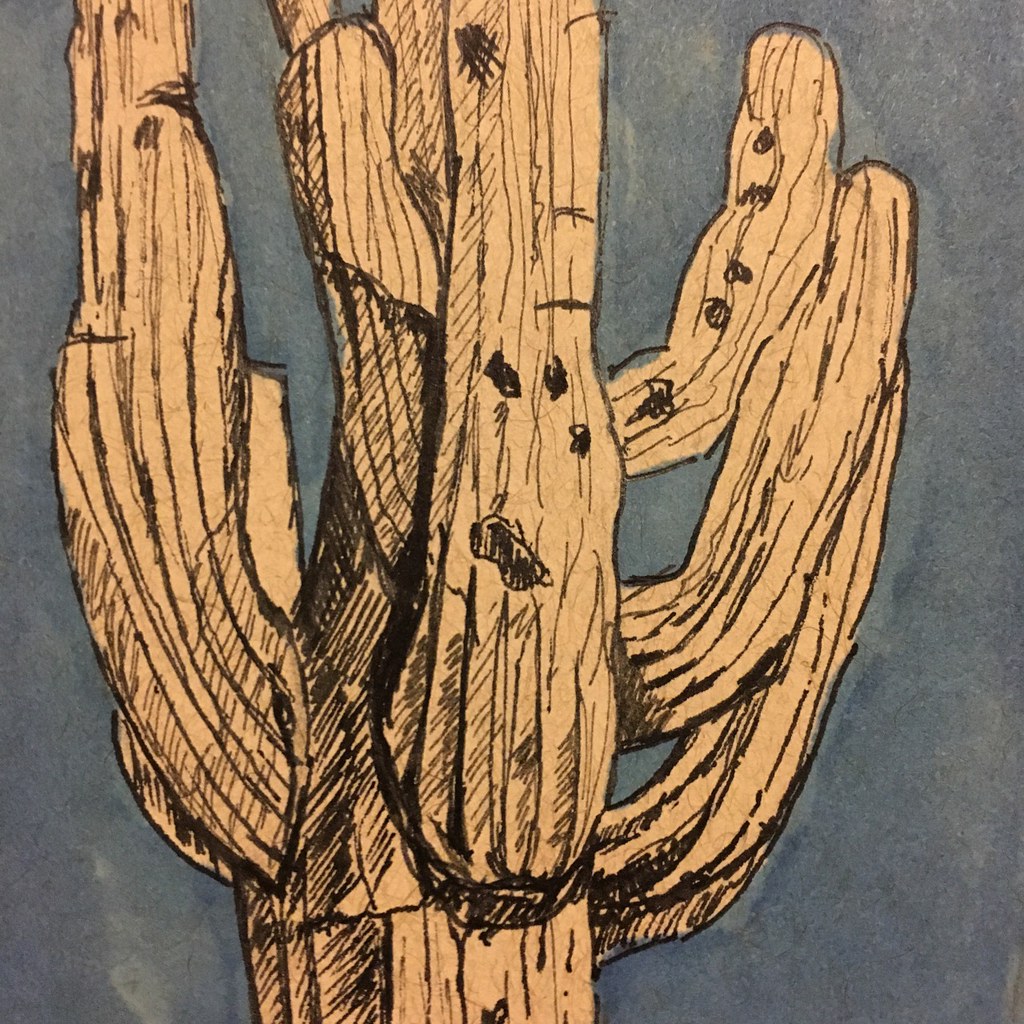This image features a digitally rendered or hand-drawn portrayal of a tall cactus set against a vibrant blue background, deviating from its typical desert habitat. The cactus is primarily beige with intricate detailing: dark black lines accentuating its contours and scattered black spots adding texture. It appears to have four to five branches extending beyond the frame, suggesting considerable height. The meticulous line work and varied shading give the cactus a striking, almost artistic presence against the contrasting sky-blue backdrop.